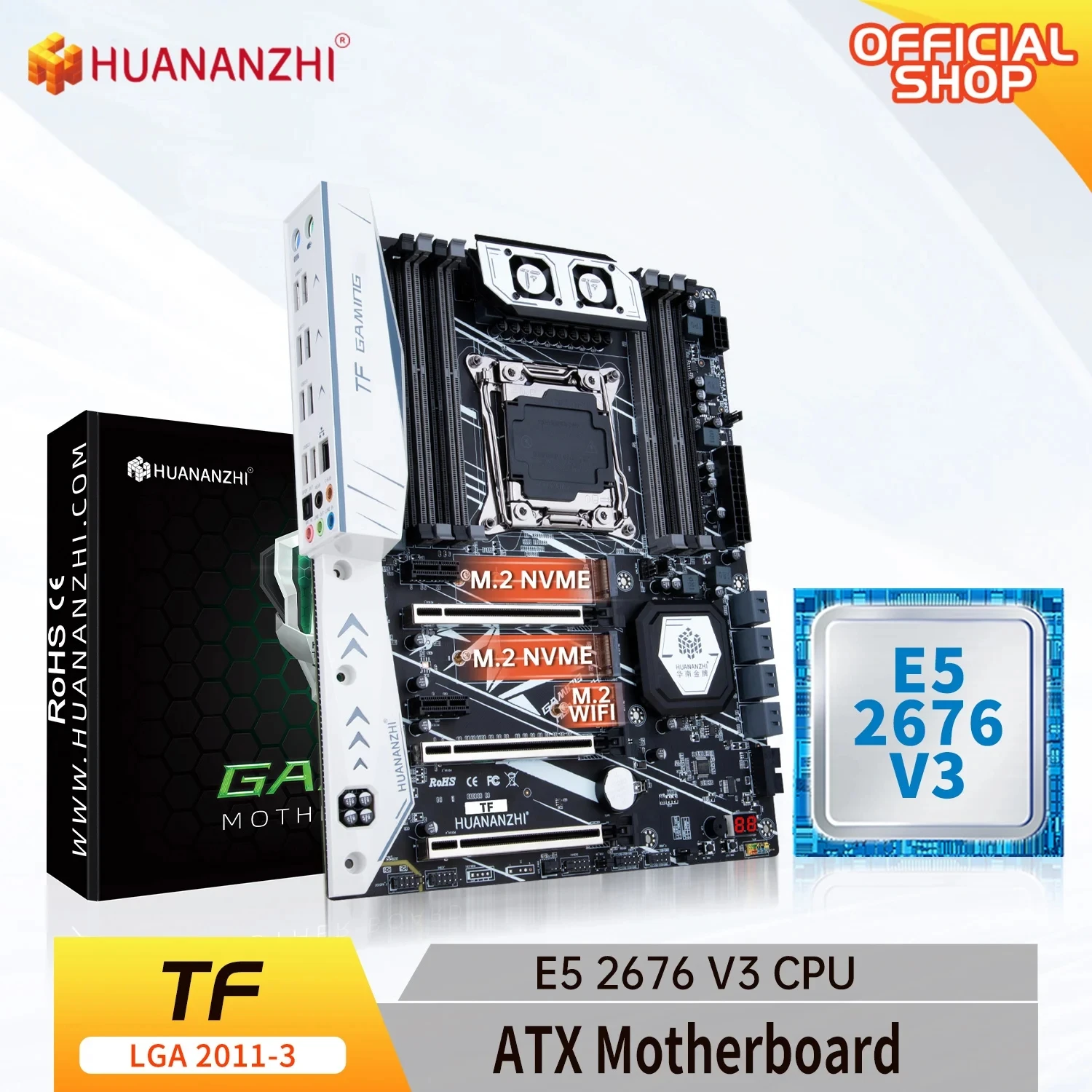This advertisement showcases an HUANANZHI ATX motherboard prominently in the center. The motherboard is visually striking with its silver and black electronic layout. On the left-hand side, there is a white panel featuring a variety of ports, including six to eight USB ports and five differently colored round ports. At the very top left corner, the brand name "HUANANZHI" is displayed in orange letters, while the top right corner features "Official Shop" outlined in orange and written in white. The image also includes a picture of the product's black and grey box, which appears on the left side. The motherboard model is indicated by bold text at the bottom, reading "E5-2676V3 CPU and TF-LGA2011-3 ATX motherboard." The board itself features numerous metal components and distinct sections, emphasizing its high-tech design and functionality. The product information also mentions "M.2 NVME Wi-Fi, www.huananzhi.com, and R-O-H-S," providing additional details about its specifications and certifications.